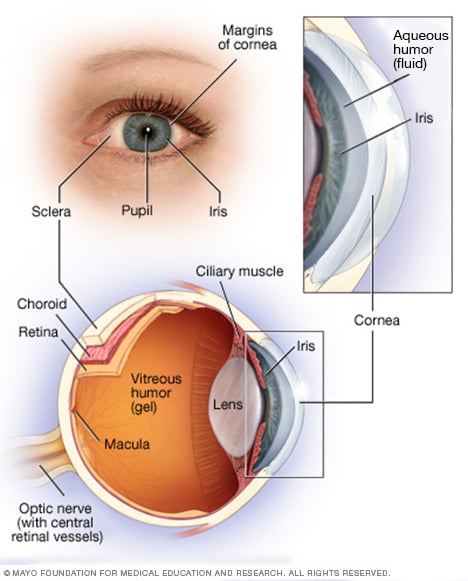This is a comprehensive, detailed digital medical illustration of the human eye, designed primarily for educational purposes, such as for medical students or aspiring optometrists. The illustration is vertically oriented and divided into three sections. 

On the top left, there's a close-up image of a blue eye, likely female, meticulously labeled with key parts such as the margins of the cornea, iris, pupil, and sclera. Adjacent to this, a smaller inset box provides a deeper view beneath the surface, highlighting important internal components like the aqueous humor fluid, iris, and cornea.

Beneath these, the bottom half of the illustration features a detailed cross-section of the entire eye. This section is thoroughly annotated, identifying the sclera, choroid, retina, ciliary muscle, iris, lens, vitreous humor gel, macula, and optic nerve with central retinal vessels. The cross-section offers an insightful look into the eye’s internal structure.

Additionally, the entire image is copyrighted at the bottom, stating that it is the intellectual property of the Mayo Foundation for Medical Education and Research, with all rights reserved. Overall, the image provides a thorough educational tool for understanding both the external and internal anatomy of the eye.